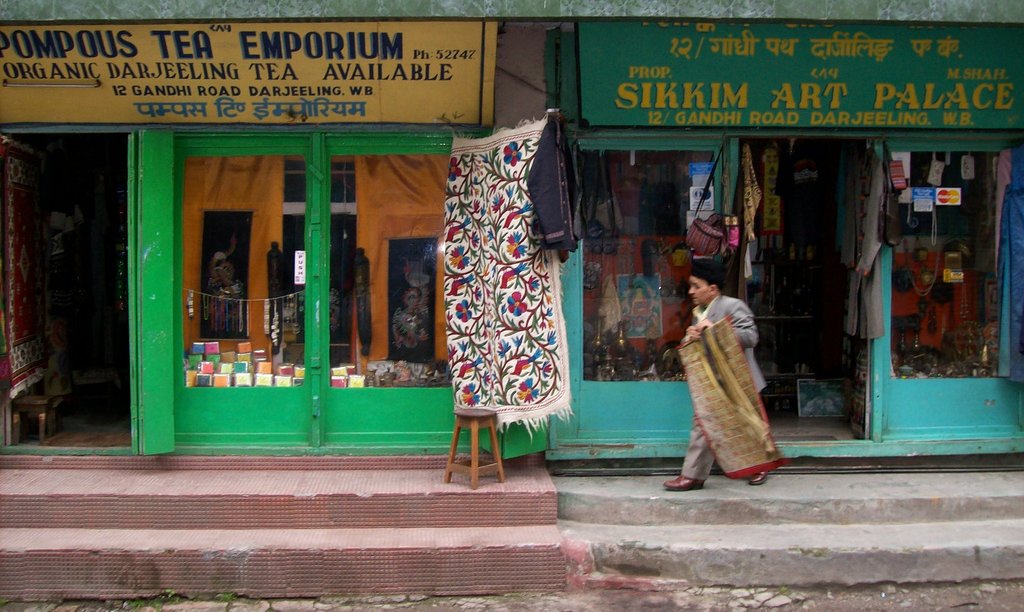This image captures a vibrant outdoor market scene in what appears to be a third-world country, with an array of colorful storefronts and intricate details. Dominating the center of the image is a short man wearing a grey suit, white undershirt, brown shoes, and a black skull cap. He carries a brownish, greenish-tan rug with red trim, walking along a crumbling, two-layered concrete sidewalk towards the storefronts.

Foreground and background elements reveal distinct details. On the left, the "Pompous Tea Emporium" features a yellow banner advertising "Organic Darjeeling Tea Available," and is located at "12 Gandhi Road, Darjeeling, West Bengal." The shop exterior is green with lighter greenish-blue highlights and contains glass display windows showcasing various tea packets and colorful items for sale.

Adjacent to it is another shop, the "Sikkim Art Palace," also located at "12 Gandhi Road, Darjeeling." This store displays a variety of traditional items, clothes, and home artifacts through its blue exterior and glass windows plastered with logos from MasterCard and other brands. Outside, a vividly designed carpet adorned with flowers and vines in blue, red, and yellow hangs beside a brown stool. The store information is displayed in both Hindi and English, naming the proprietor as Mohammed M. Shah.

The scene is awash with colors including pink, tan, green, black, white, blue, red, maroon, orange, yellow, and light blue, enhancing the bustling atmosphere of a midday market.